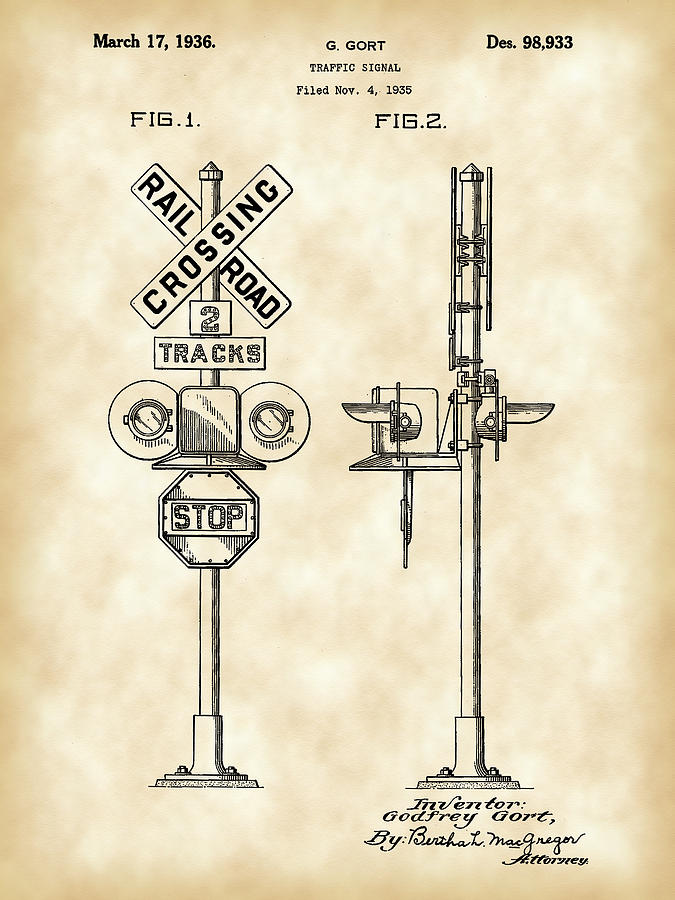This detailed, black-and-white diagram of a railroad traffic signal appears on a piece of parchment-like paper with gold-toned, worn edges and brown discoloration, giving it an aged appearance. At the top left corner, the date "March 17, 1936" is prominently displayed in black letters. Centrally located at the top, the text reads "G. Gort, Traffic Signal, Filed November 4, 1935," while the top right corner features "DES 98,933."

The diagram is labeled with two figures: Figure 1 on the left and Figure 2 on the right. Figure 1 illustrates a traditional railroad crossing sign. It shows a crossbuck sign that spells out "RAILROAD CROSSING," mounted on a metal pole that is bolted to the ground. Underneath this crossbuck, there is a sign with the number "2," followed by another sign that says "TRACKS." Below these, a circular signal light setup, separated by a square box likely housing the battery or bell for alerts, is depicted. At the bottom of this assembly, an octagonal stop sign with the word "STOP" across the center is featured.

Figure 2 presents a side view of the same railroad crossing setup, detailing how the various components – including bolts, fasteners, lights, and signs – are mounted to the pole and flange that anchors the structure to the ground. This side view facilitates understanding the construction and assembly of the traffic signal.

Beneath Figure 2, the image credits the inventor, stating "Inventor: Godfrey Gort, by Bertha L. McGregor, Attorney," written in a script font. The entire instructional sheet showcases detailed engineering and design specifications for a railroad traffic signal, intended for manufacturing and practical use.